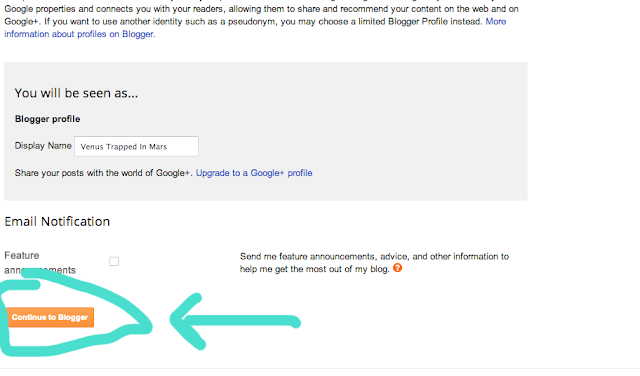On a crisp white background, the image is segmented into several distinct sections, primarily in black and blue text. At the top, in black font, it reads "Google Properties," and then continues in smaller text, explaining its purpose: "connects you with your readers, allowing them to share and recommend your content on the web and on Google+". 

Below this, the document provides an option for identity choices. It states: "If you want to use another identity, such as a pseudonym, you may choose a limited blogger profile instead." Beneath this explanation, a prompt with blue font reads, "More information about profiles on Blogger."

A gray background text box then appears with the message: "You will be seen as..." followed by the bold text, "Blogger Profile Display Name". Adjacent to this, there is a white text box where users can enter their desired display name. In this instance, it is filled with the name "Venus Trapped in Mars".

Further down, it suggests sharing posts by stating: "Share your post with the world of Google+," followed by an actionable call-to-action in blue clickable link text: "Upgrade to Google+ Profile."

There is also a section regarding email notifications, with a checkbox for "Feature Announcements" that is unchecked. The accompanying text reads: "Send me feature announcements, advice, and other information to help me get the most out of my blog."

At the bottom, there is a prominent orange button labeled "Continue to Blogger" in white text. This button is visually emphasized with an aqua-colored circle around it and an aqua-colored arrow pointing towards it, seemingly photoshopped for additional emphasis.